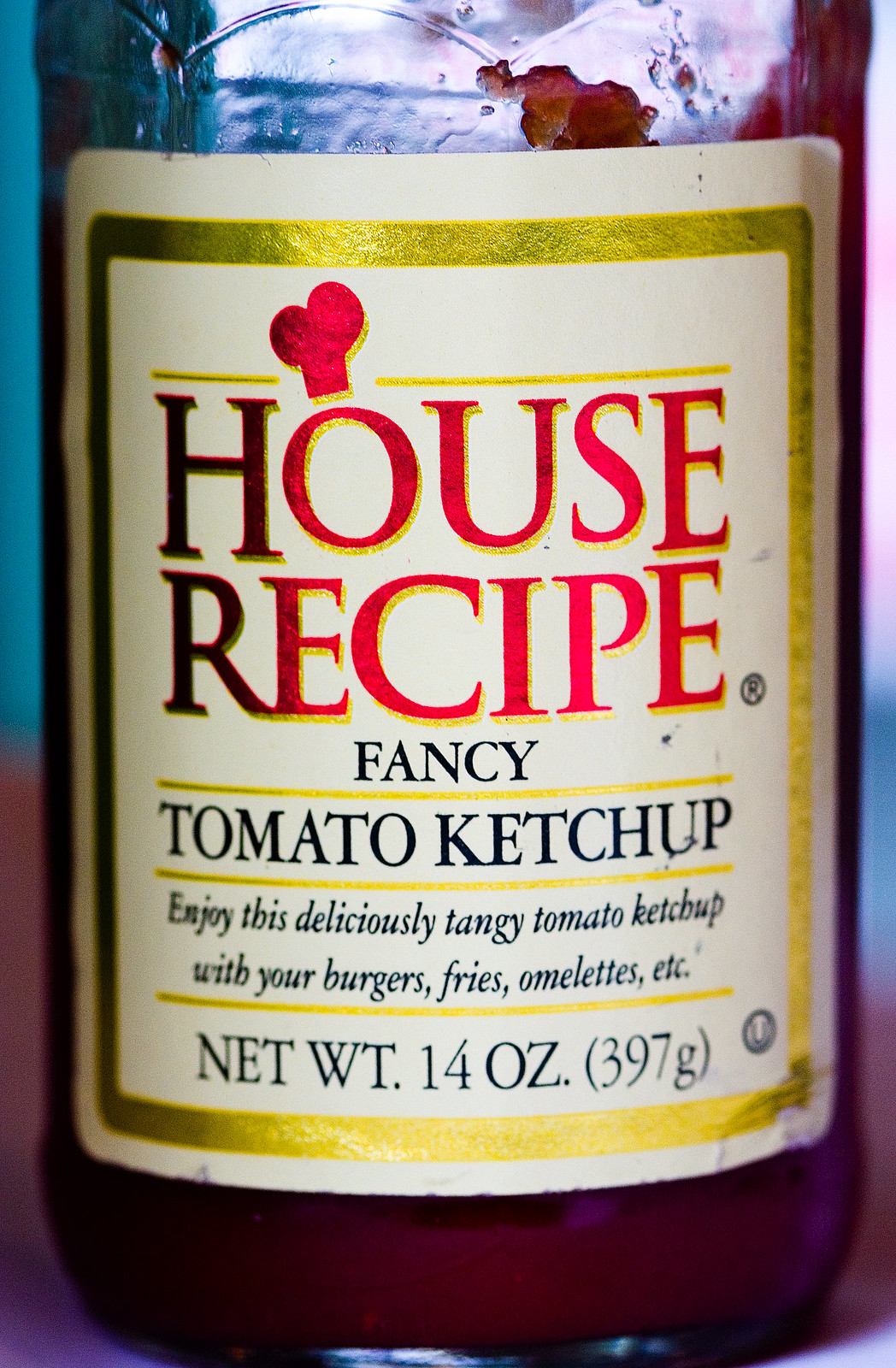This photograph depicts the bottom half of a clear glass ketchup bottle, filled about a third to half with rich, red ketchup. Some of the ketchup is slowly sliding down the inner surface of the bottle. The bottle features a distinctive white label with a gold border. Prominently displayed in red text on the label is the brand name "House Recipe," with a chef's hat adorning the "O." Below that, in black text, it reads "Fancy Tomato Ketchup." The label also includes a description: "Enjoy this deliciously tangy tomato ketchup with your burgers, fries, omelets, etc." The net weight of the ketchup is listed as 14 ounces (397 grams). The bottle sits on a whitish table, casting a subtle shadow, with a slight glare from the lighting. The bottom right-hand corner of the label appears a bit worn, indicating it has been well-used. The edges of the image have a hint of a blue background.